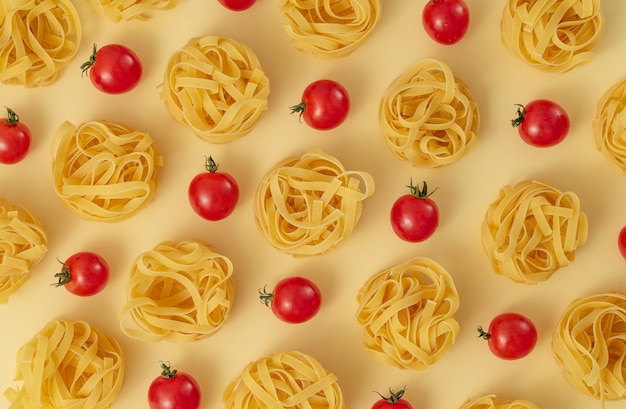This image showcases a meticulously arranged food display that could be ideal for a food blog, website, or menu. It features neat circular patterns of yellow, wavy fettuccine noodles, interspersed with rows of round, juicy red cherry tomatoes. The layout is set in alternating diagonal stripes, with pasta circles and tomatoes creating a visually appealing sequence. The background is a light beige or off-white color, suggesting a modern kitchen counter or a butcher block. Shadows cast by the pasta and tomatoes add depth to the composition, enhancing the overall aesthetic appeal.